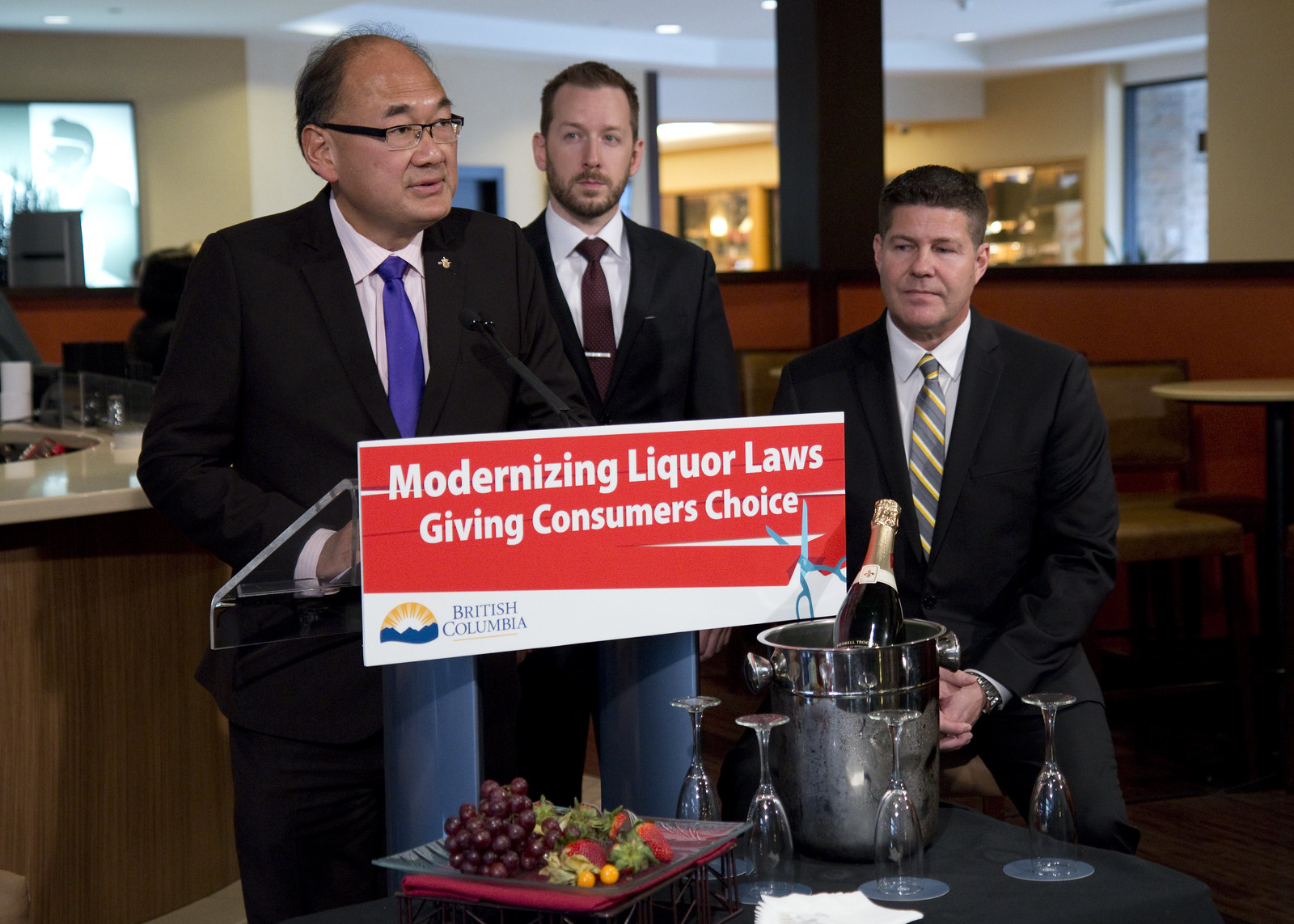In this horizontally aligned, rectangular image, three men are positioned behind a table within what appears to be a restaurant setting. The restaurant features booths to the right, yellow walls in the background, and white ceiling with recessed fluorescent lighting. Behind the men, there is a bar with a wooden base and a black top, and a TV screen is visible in the background.

These men, all dressed in dark suits, stand together. The first man, positioned at a podium and speaking into a microphone, is an older Asian man with balding hair and short black hair on the sides. He wears dark-framed glasses and a blue tie. In front of his podium is a sign that reads "Modernizing Liquor Laws, Giving Consumers Choice," with the lower left corner bearing the text "British Columbia." Directly in front of the sign, there is a stainless-steel bucket holding a bottle of champagne, surrounded by upside-down wine glasses, and a platter with grapes and strawberries.

The second man, standing in the middle, is younger with dark hair, a short beard, and a mustache. He wears a dark red (or burgundy) tie and a white shirt, and directs his attention towards the speaker.

The third man, on the right, appears to be in his 40s with dark hair. He wears a blue and yellow (or gray and yellow) striped tie and also a white shirt. All three men are standing behind a table covered with a black cloth.

The restaurant's ambiance, although slightly blurry in the background, reveals a comfortable and decorated environment suitable for formal events or press conferences.